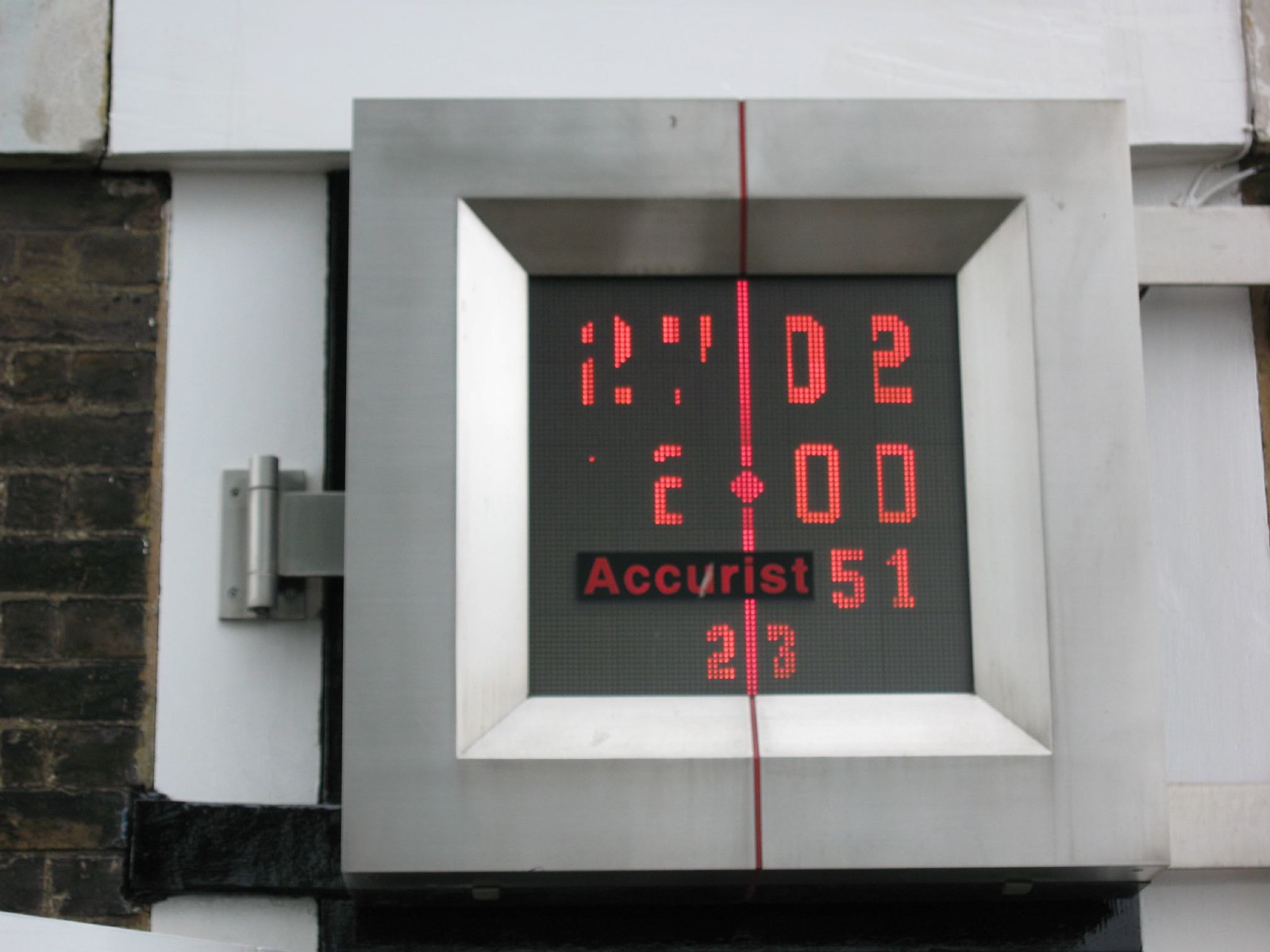This horizontal color photograph presents a detailed view of a large metal square fixture, possibly the side of a building, prominently featuring a digital display. The metal square, secured with a metal bracket underneath and potentially designed to open via a visible metal hinge on the left, is characterized by an inset screen displaying red lit-up numbers and letters against a black background. At the very top of the screen, the number "2702" is visible, followed by red letters "E," "O," and "D" arranged in a sequence across the middle. Below these characters, the word "Accurist," spelled out as A-C-C-U-R-I-S-T, is clearly visible in red at the bottom third of the screen. Additionally, the numbers "51" and "23" are also visible amidst the red digital display. The fixture is bisected vertically by a red line, which appears either as drawn or illuminated in segments, running from the top center, through the screen, to the bottom. Surrounding the central square, the photograph captures elements of its setting: a dark-colored brick wall on the left side, contrasted by white beams or metal painted white above, creating a structural backdrop for this enigmatic digital display.